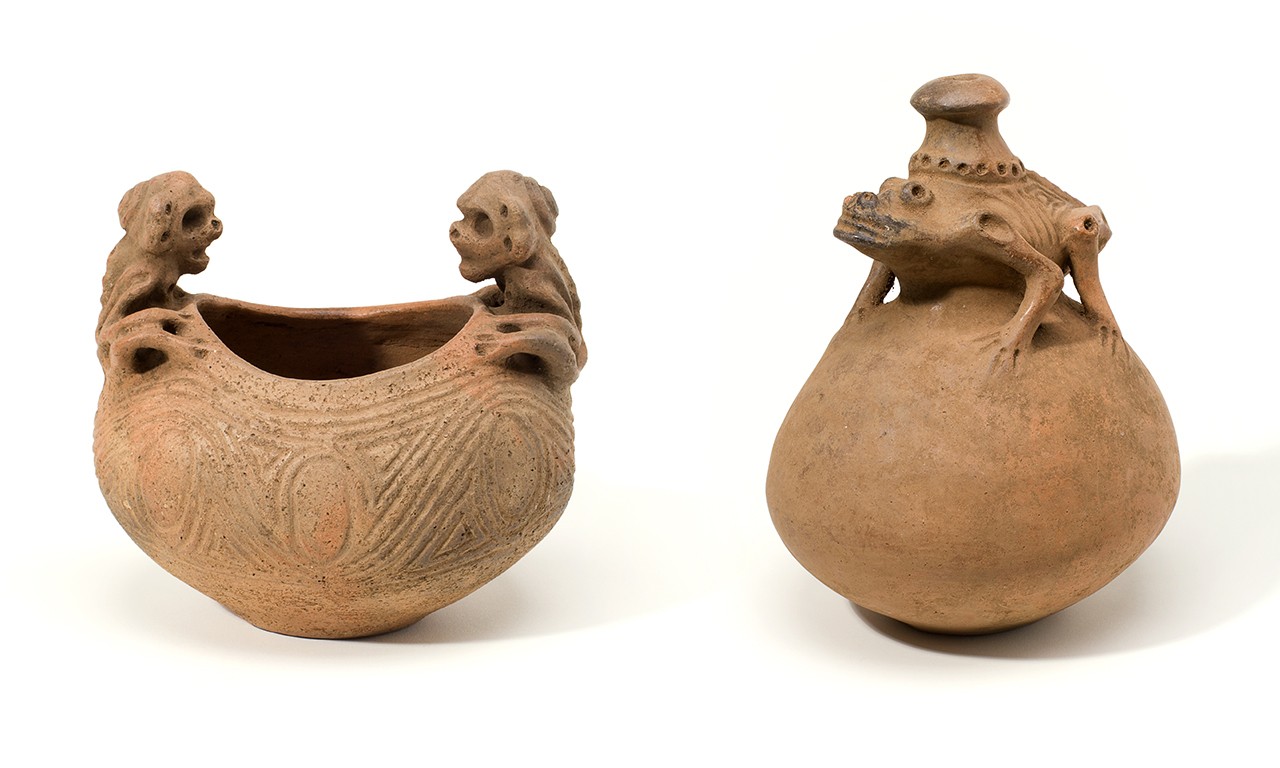The image showcases two ancient-looking wood-carved pottery pieces, set against a plain white background, emphasizing their intricate details and likely their historical significance. Both pieces share a light brown, beige coloration, suggesting they might be made from similar material, possibly clay. The more detailed bowl on the left is hollow and features two skeletal, monkey-like creatures with open mouths, perched on its rim, possibly roaring at each other. Their crouched, four-legged stance enhances the bowl's overall menacing yet artistic vibe. This piece, oval in shape, also includes etched lines and three oblong decorations around its surface, highlighting its craftsmanship.

Beside it, the second sculpture features a spherical base and is topped with a frog-like creature with four limbs, belly-down as if resting on the ball. The frog has a protruding knob from its back, giving it an added dimension or functionality, potentially as a lid or handle. This piece, more closed in design compared to the first, exudes a sense of completeness. Both artifacts likely have significant cultural symbolism, possibly hinting at their origins from ancient civilizations such as the Incas, Mayans, or Egyptians, making them fitting for a museum exhibit.